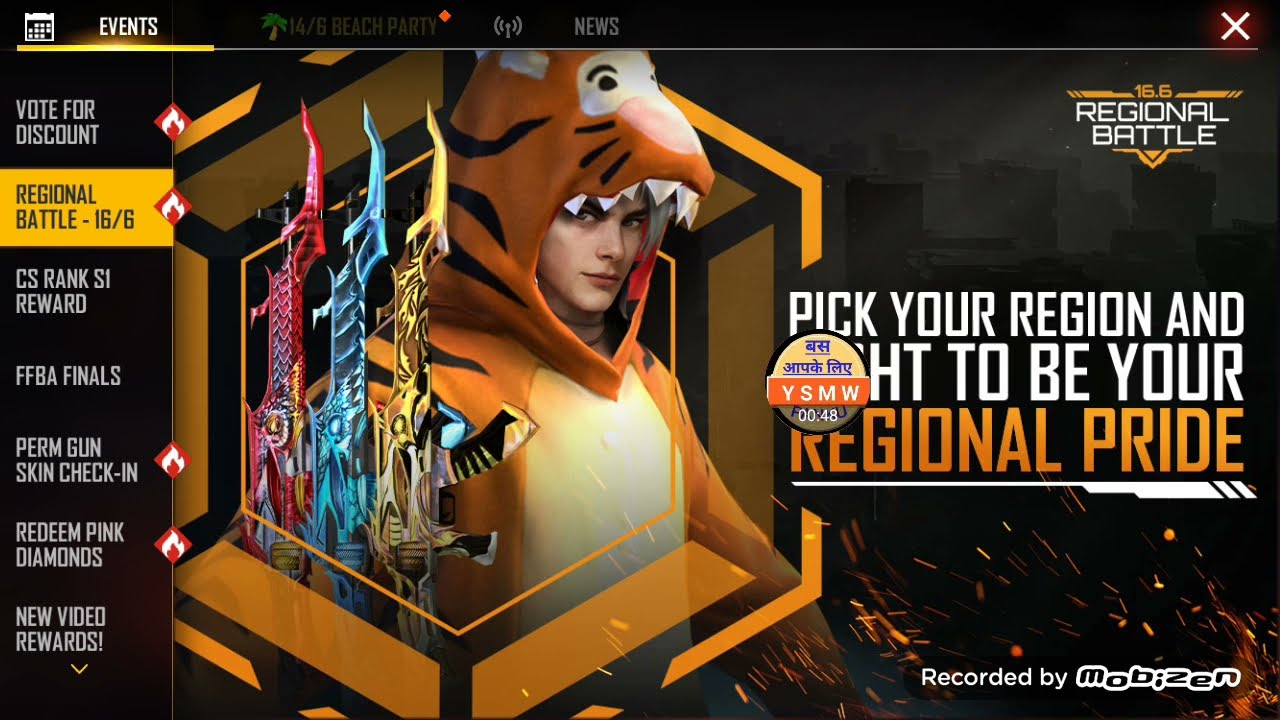The image appears to be a screenshot from a video game menu screen. The background is predominantly black, scattered with fiery sparks towards the bottom right. Text elements are dispersed across the screen. In the upper right corner, a horizontal menu includes an "X" button and the text "16.6 Regional Battle." Below, it instructs, "Pick your region" and another line partially obscured reads, "fight to be your regional pride," with "regional pride" highlighted in orange letters. Dominating the center is a character donned in a tiger suit, through whose open mouth the character's head and face are visible. Surrounding the character are vibrant, yellow-orange graphics and three colorful weapons—a red, a blue, and a yellow assault rifle, each adorned with curved bayonets. To the left edge of the image, a vertical menu lists game options. Text in the top left corner mentions various game events and rewards, including "vote for discount," "CS rank C reward," and "FFBA finals perm gun skin." The bottom right corner features the recording credit: "Recorded by Moby Zen."